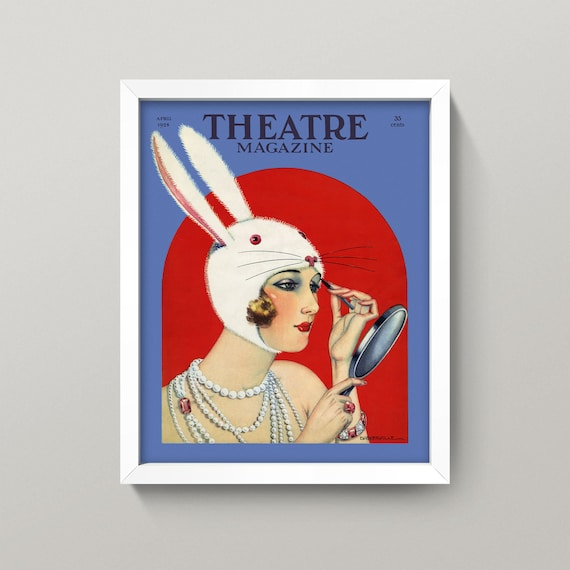This image showcases a framed magazine cover titled *Theatre Magazine*. The white frame surrounds a vibrant piece of art that embodies the aesthetic of the 1920s. Central to the cover is a flapper girl adorned in a distinctive rabbit hat complete with realistic eyes, ears, nose, and whiskers. She is immersed in applying her makeup, holding a handheld mirror in her left hand while delicately painting her eyebrows with a pencil using her right hand. Her look is accessorized with multiple strands of pearl necklaces, a jewel-encrusted bracelet on her right wrist, and a gem ring on her left hand. The background of the magazine cover contrasts boldly with a light blue surrounding and a red arch framing the woman. Text on the top left corner indicates "April 1920," while the top right corner, though slightly blurry, shows the price of "35 cents." This detailed artwork captures a moment of personal grooming, set against a vibrant and graphical blue and red color scheme.